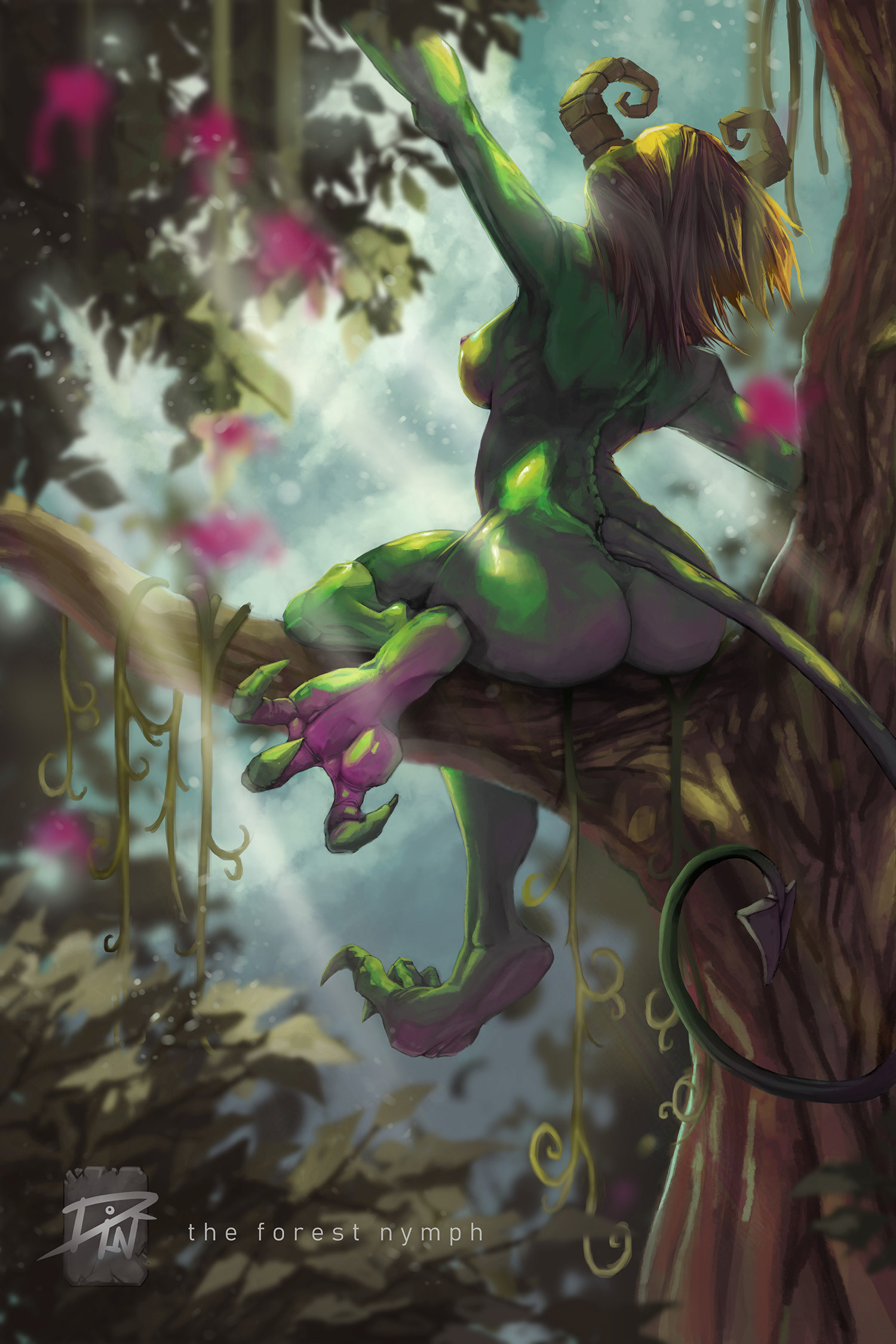In this detailed, animated art piece titled "The Forest Nymph," we see a mystical, humanoid female creature blending elements of both woman and mythical being. The nymph, with her greenish skin and flowing green hair, is perched gracefully on a horizontal branch that spans the middle of the image. This branch extends from a tall, light brown tree rising along the right edge of the picture, adorned with green vines and pink flowers. The lush, mystical forest background is illuminated by dappled light shining through the foliage, adding an ethereal glow to the scene.

The forest nymph is depicted from the back, slightly turned to the left, her large posterior and exposed breasts visible as she sits on the branch. Her body exhibits exotic features: a long tail with a triangular point curling around her, large feet with three pronounced claws, and two prominent, curled horns on her head. She appears to be stretching or yawning, her arms extended outward. Accentuating her otherworldly beauty, her hair cascades just past her shoulders in a blonde hue with green undertones.

At the bottom of the image, in white text, is the title "The Forest Nymph," accompanied by a gray logo on a rectangular background that reads "din din." This artwork, rich with shades of green and pink, captures the enchanting essence of the mythical forest and its mysterious inhabitant.